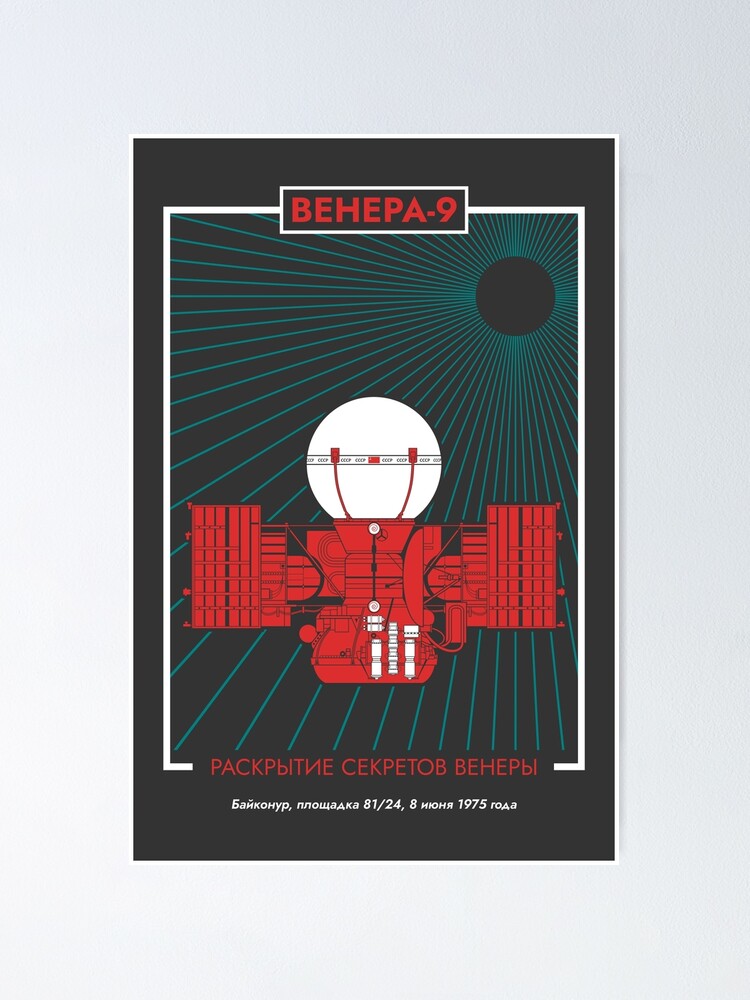The image is a digital art poster featuring a primarily black background with a solid black border and a white glowing orb in the center. At the top of the poster, the title "BEHEPA-9" is prominently displayed in red, while the bottom of the poster contains text in Russian, "ПЕКТИК СИПЕТОП БЕВИПИ," followed by a smaller subscript in white. In the upper right of the image, a black eclipse-like sphere emits teal-colored rays that spiral outward, intersecting with a futuristic red mechanical contraption centrally depicted. This contraption appears to be an intricate device with interconnected red structures, resembling a satellite with a large white halogen light bulb held by two red prongs at its peak, akin to a desk lamp bulb. The apparatus also features panels and beams, and a jet-engine-like component at its base. The poster is mounted on an off-white colored wall, enhancing its striking visual contrast.